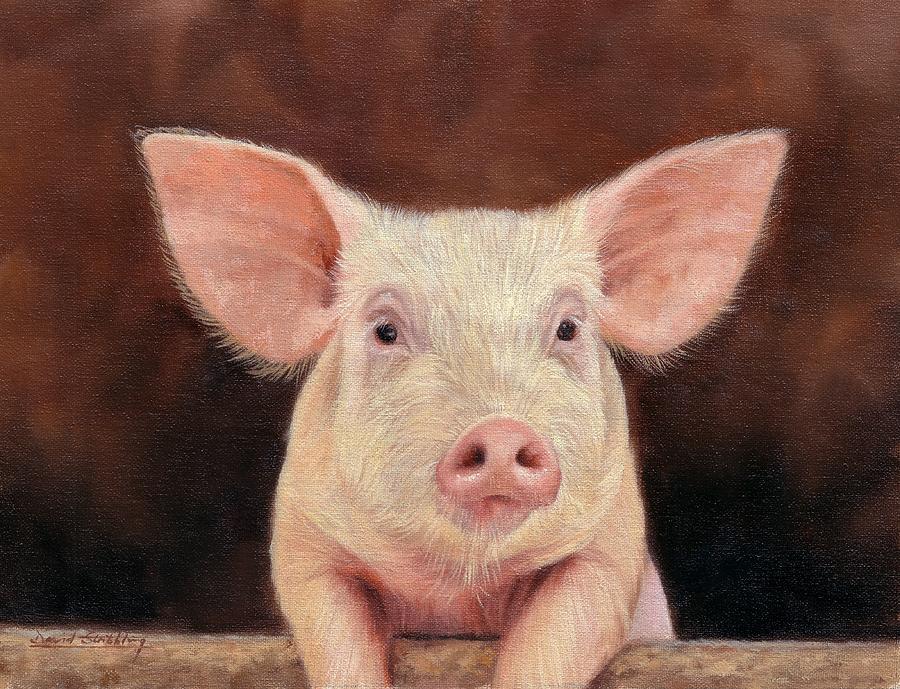In this image, we observe a beautifully detailed painting of a piglet, depicted from the shoulders up, with its front legs draped over what appears to be a piece of wood or a log. The little piglet is painted with a blend of pinks and creams, giving it a soft, lifelike appearance. The face is framed by large, alert ears - pink on the inside and pale cream on the outside - and covered in light, white fur. The piglet gazes directly ahead with small, black eyes and a sweet expression, complemented by a characteristic pink snout. Behind the piglet, the background features a gradient of dark to medium browns, becoming darker towards the bottom. A small signature in the bottom left-hand corner reads 'David,' followed by an unclear last name and a tiny date. The slight shininess in the top corner suggests that this is likely an oil painting.